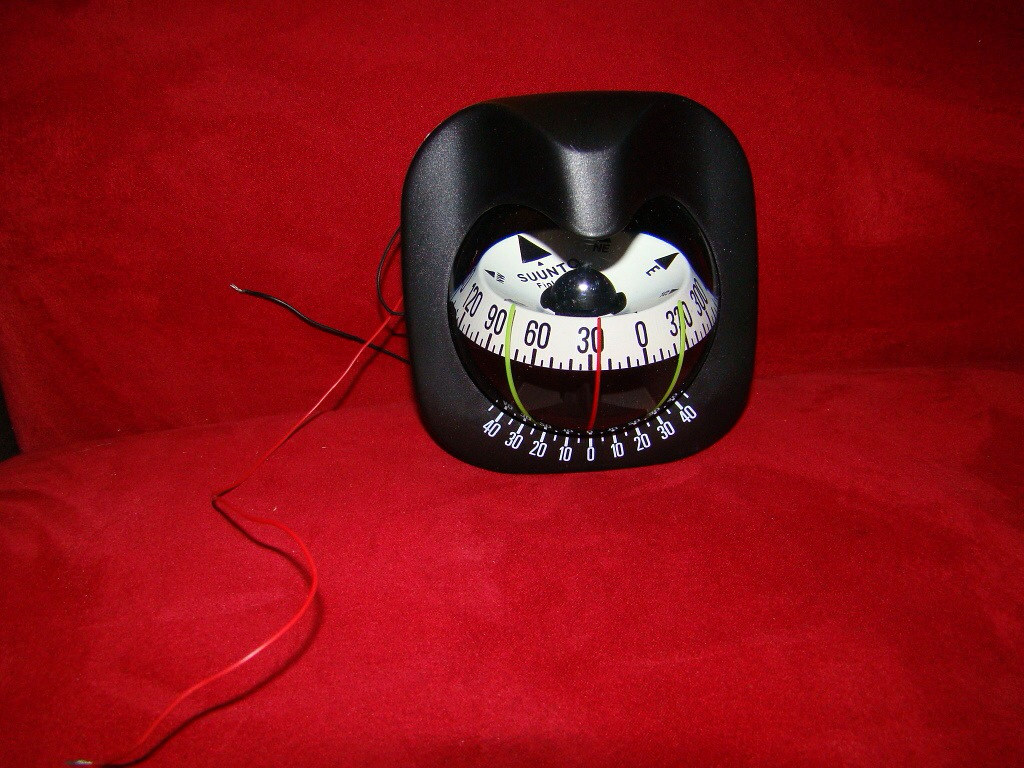The photo features a rich, red velvet background that extends from the lower half to the upper portion of the image. The texture indicates it's a soft fabric. In the middle left of the photo, where the red fabric's lines meet and extend upwards, there is a subtle darkening, perhaps indicating the edge of the backdrop.

Centrally positioned is a black mechanical device, somewhat reminiscent of a sundial. From this device, a red wire snakes off to the bottom-left corner in a gentle S-curve, terminating at the edge of the frame. Additionally, a black wire extends approximately two inches from the left side of the device, where it abruptly ends. Adjacent to this wire, there is an indistinct loop of black material, possibly related to the black wire but it's not clearly connected.

At the bottom of the black device is a dial with a scale ranging from -40 to 40, with a green bar on the left at -40, a red bar at the midpoint of 0, and another green bar at the right end of 40. This dial appears to lead up to a curved section holding a spherical object. The top part resembles a bowl with the sphere resting centrally. Markings around this sphere range from 120 to 300, accompanied by directional arrows indicating north, east, and south. The black device holds and points towards this central sphere, suggesting it is secured or controlled by it.